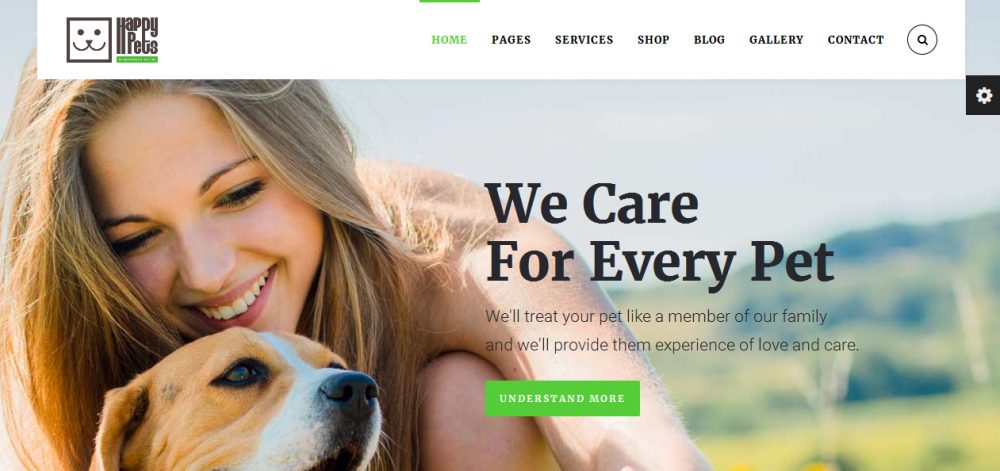This image is a screenshot from a pet care website. The upper left-hand corner features a cute square icon with a joyful dog face, labeled "Happy Pets." Centered at the top of the page are navigation tabs including Home, Pages, Services, Shop, Blog, Gallery, and Contact, along with a magnifying glass for search functionality. The Home tab is highlighted in green, indicating it is the current page. In the upper right corner, a cog icon suggests settings or customization options.

Dominating the image is a heartwarming photo of a blonde woman happily smiling with her brown dog, which has a white snout. Overlaid on this image, in bold black letters, is the phrase "We Care for Every Pet." Beneath that, in smaller text, it reads, "We'll treat your pet like a member of our family and provide them experience of love and care." At the bottom of the image, there is a green rectangular button with the text "Understand More."

The overall design and content emphasize a welcoming and care-centered approach to pet care, aimed at assuring pet owners of the love and dedication their pets will receive.